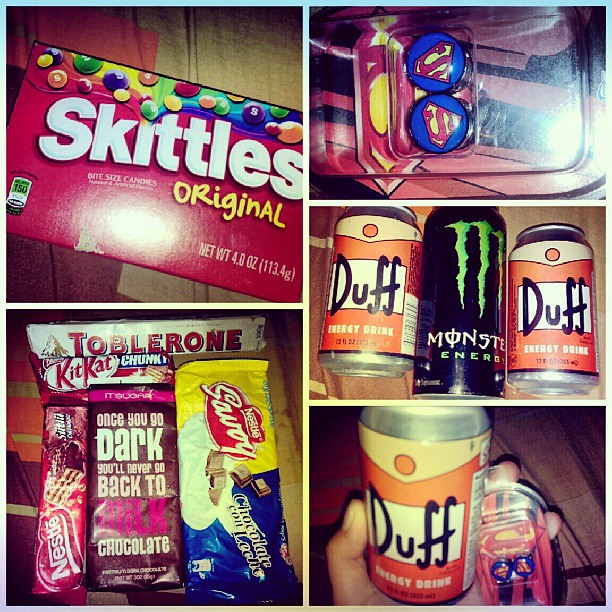This image features a collage of five different photographs showcasing a variety of snack foods and items. In the top left, there's a box of Skittles Originals, vibrant with its standard red packaging and bite-sized, multi-colored candies. Below that, the bottom left image displays an assortment of chocolates, including a Toblerone bar, a Kit Kat Chunk, a Nestle Savoy bar with the tagline "Once you go dark, you'll never go back to milk chocolate", and another unnamed chocolate bar. Moving to the right side, the top-right section contains two blue badges with the iconic Superman logo. Just below, in the middle-right, are two cans of Duff Energy Drink flanking a can of Monster Energy Drink. Lastly, the bottom right photograph captures another view of the Duff can alongside the Superman logo badges. The layout consists of evenly spaced objects, creating an organized but eclectic collage of colorful snacks and memorabilia.